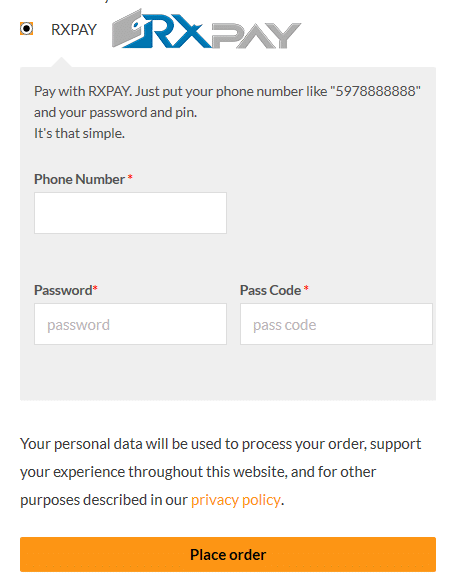This image appears to be a screenshot of the login page of a website or mobile app named RxPay. At the very top center, the title "RxPay" is prominently displayed, with "Rx" in blue and "Pay" in gray. 

In the main section of the page, users are prompted to input their phone number, password, and passcode. There is a brief description that reads, "Pay with RxPay. Just put your phone number, like '597-888-8888', your password, and PIN. It's that simple." 

Toward the bottom of the screen, there is another description explaining the use of personal data: "Your personal data will be used to process your order, support your experience through this website, and for other purposes described in our privacy policy."

At the very bottom, there is a long, rectangular, orange button centered in the screen with the words "Place Order" in black font.

This comprehensive login interface provides users with straightforward instructions and clearly conveys how their information will be utilized.